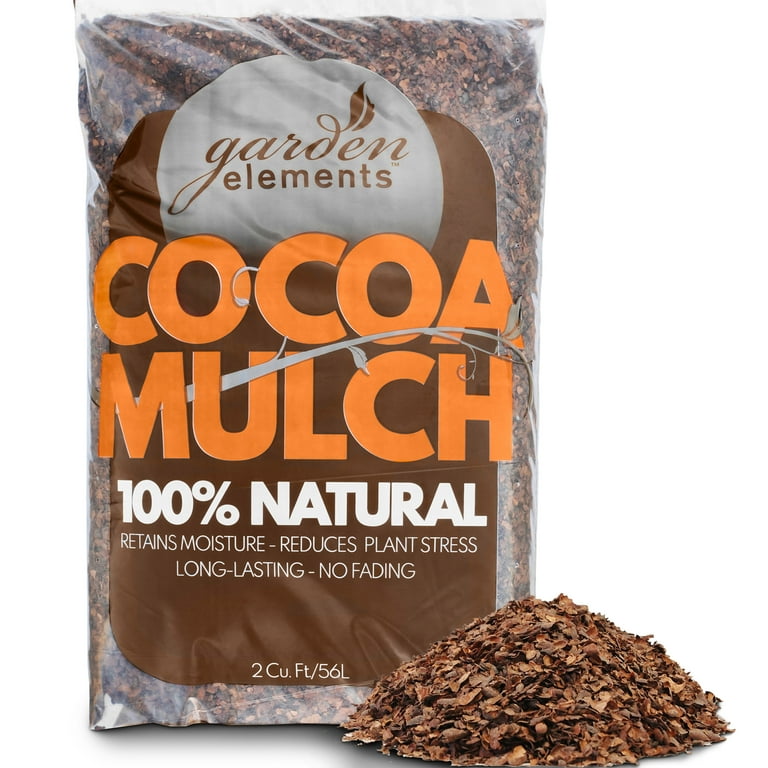This product image showcases a bag of cocoa mulch in its packaging, prominently displaying the brand name "Garden Elements" in a circle at the top. The "cocoa mulch" text is featured in large, vibrant orange letters with a tree branch weaving through the 'U.' The packaging highlights key benefits with bold text stating "100% natural," "retains moisture," and "reduces plant stress." The label further emphasizes the product's longevity with claims of "long-lasting" and "no fading." The bag details the quantity as "2 cu feet / 56 liters." In front of the bag, a small cone-shaped pile of mulch illustrates the product’s texture and appearance. The overall design includes a combination of cursive and block lettering on a predominantly brown background, giving the packaging an earthy and natural feel.